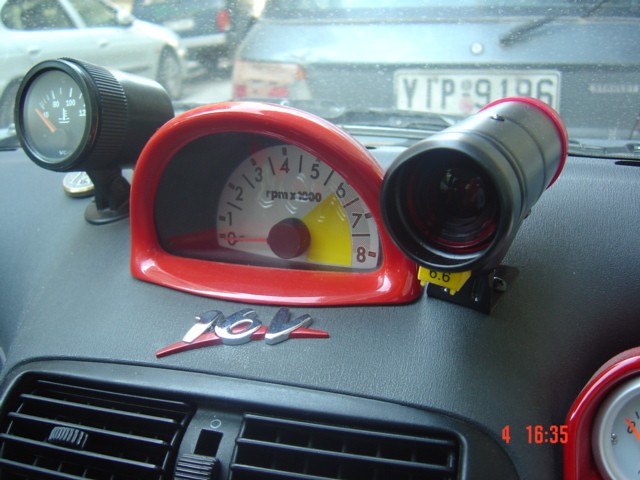In this image, we observe the intricate interior of a car dashboard, prominently displayed at the bottom right corner. A digital overlay showcases a red number "4" followed by "16:35," indicating the time or a specific reading likely added by the camera. Centrally positioned, a striking semi-circular red console commands attention. Its design features a flat bottom and a prominent, thick, lip-like border. Resting within this bold console is a prominent white dial labeled "RPM x 1000," with numerical indicators ranging from 0 to 8. The dial becomes particularly eye-catching from the number 6 onwards, where it is filled in with a vivid yellow shade.

To the left of this main console, there's a smaller gauge, likely for temperature, displaying a scale from 0 to 120 or 125. On the right side, an unusual object resembling a telescope with a central glass component suggests it might be another gauge or possibly a camera, though its exact function remains ambiguous. Below these elements, air vents are visible, contributing to the dashboard's functionality. Above the entire arrangement, the text "16V" is elegantly scripted in chrome, accompanied by a sleek red graphic resembling a banana underneath, which adds a stylistic flair to the ensemble.